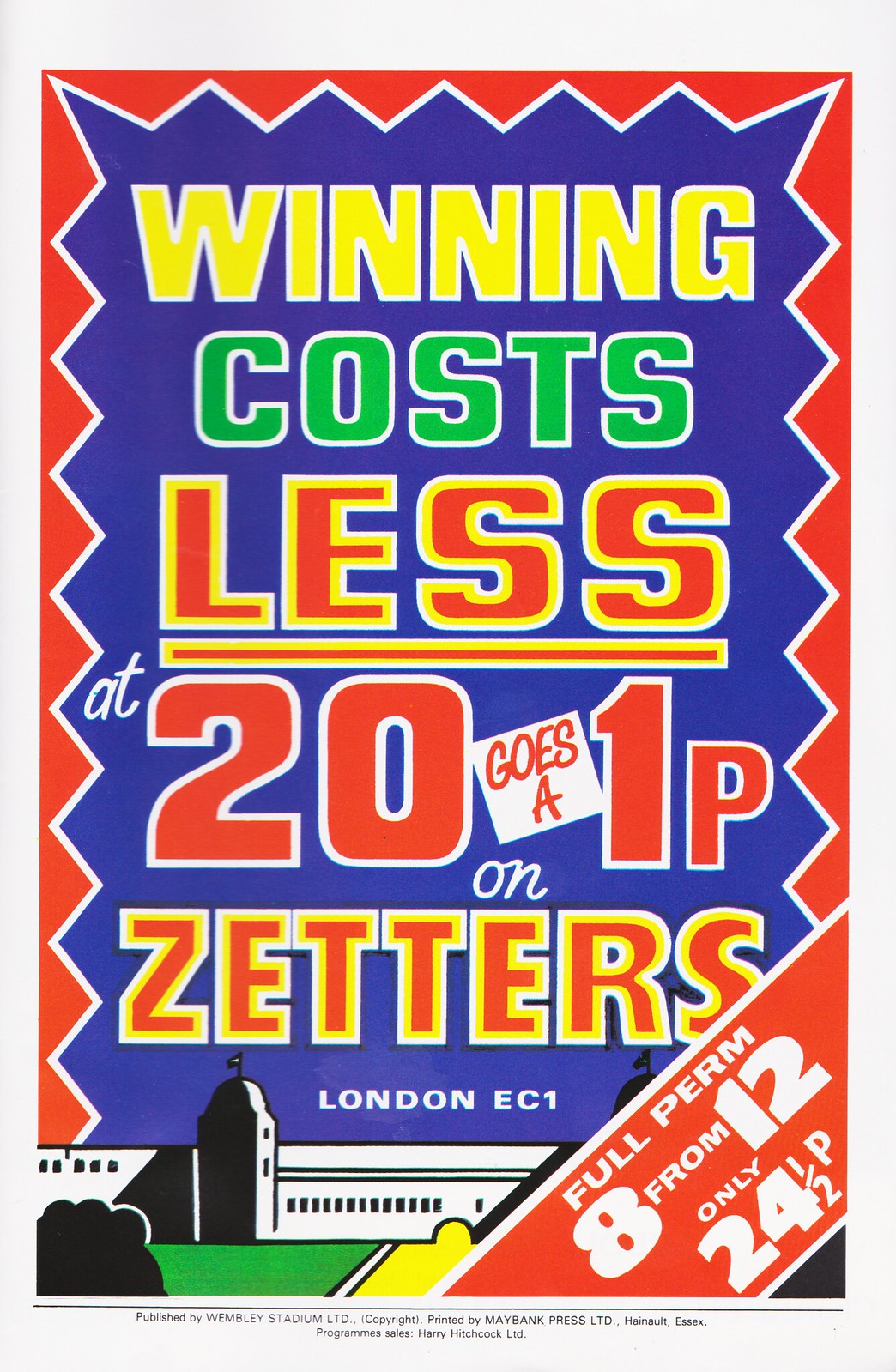The image is a detailed graphic flyer designed with vibrant colors and various elements. It features a light gray border along the top and sides, encapsulating a vivid rectangular design. The outer edges of the flyer are swathed in red, transitioning to a blue background in the center. Intricately placed squiggly lines and pointed triangles emanate from the red border, adding a dynamic touch to the visual.

Dominating the top of the blue section, the word "WINNING" stands out in bold yellow capital letters, outlined in white. Directly beneath, the word "COSTS" appears in green, also edged with white borders. Following this, the word "LESS" is presented in striking red with contrasting yellow and white outlines. Below these primary statements, a red line stretches horizontally.

To the left side of this line, in small white letters, the word "AT" can be seen. Adjacent to it, the number "20" is prominently displayed in large red digits, followed by the text "GOES A" in a small white box. Next to this, the number "21P" appears in red, emphasizing the price.

Further down, the word “ON” is written in white letters, succeeded by "ZETTERS" in bold red text. Below this, in smaller white print, "London EC1" provides a hint at the location. 

The lower section of the flyer features an image of a building extending from the left to the right edge until interrupted by a diagonal red banner. This banner carries the words "FULL PERM" and continues with the text "8 FROM 12," followed by "ONLY" and "24 AND A HALF PENCE," arranged at an angle from left to right. Beneath the main poster, there are a few lines of very small black print that finalize the intricate design.